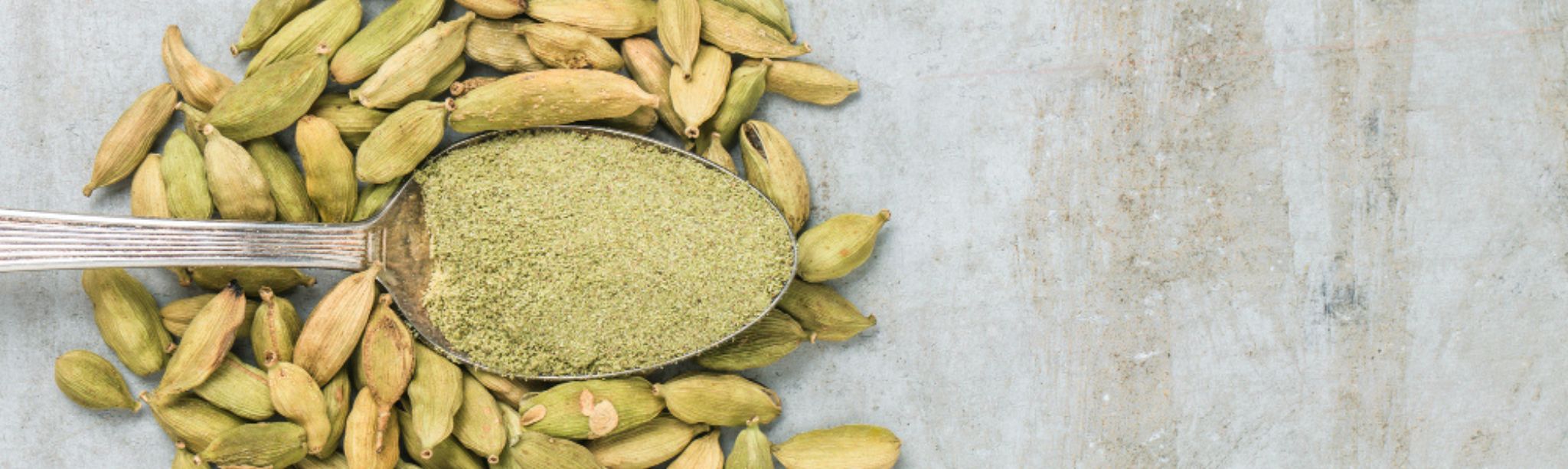The image showcases a tarnished silver spoon filled with a greenish-yellow granulated powder, resting on a pile of small, oval-shaped, greenish-brown seeds or pods. The handle of the spoon extends out of the frame to the left, featuring grooves or ridges along its length, while the spoon itself is positioned to the right. The seeds surrounding the spoon vary in color from beige to green and resemble small nuts or pumpkin seeds. The whole scene is set on a gray and brown mottled surface, possibly a concrete table or a stained marble countertop. The image is a top-down shot, emphasizing the contrast between the green powder in the spoon and the mixed-color seeds below.